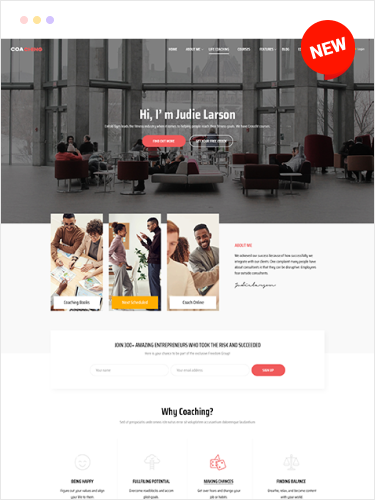Screenshot of Judy Larson's home page from her coaching website. The header features a white banner adorned with pale pink, yellow, and purple spots, likely serving as the navigation menu. In the top left corner, partially obscured text possibly reads "COA COLE" and "CHINO" among other options. The right-hand side of the banner presents more navigation options such as "Home," "About," "About Me," and more, though the exact words are difficult to decipher.

Prominently displayed is a large red circle with white capital letters stating "NEW," though the specifics of the novelty are unclear. Below, the text introduces Judy Larson, although the subtitle is illegible. Another visible section titled "Why Coaching?" suggests the website's focus on lifestyle coaching. The background image depicts what appears to be an office space, adding a professional ambiance to the site.